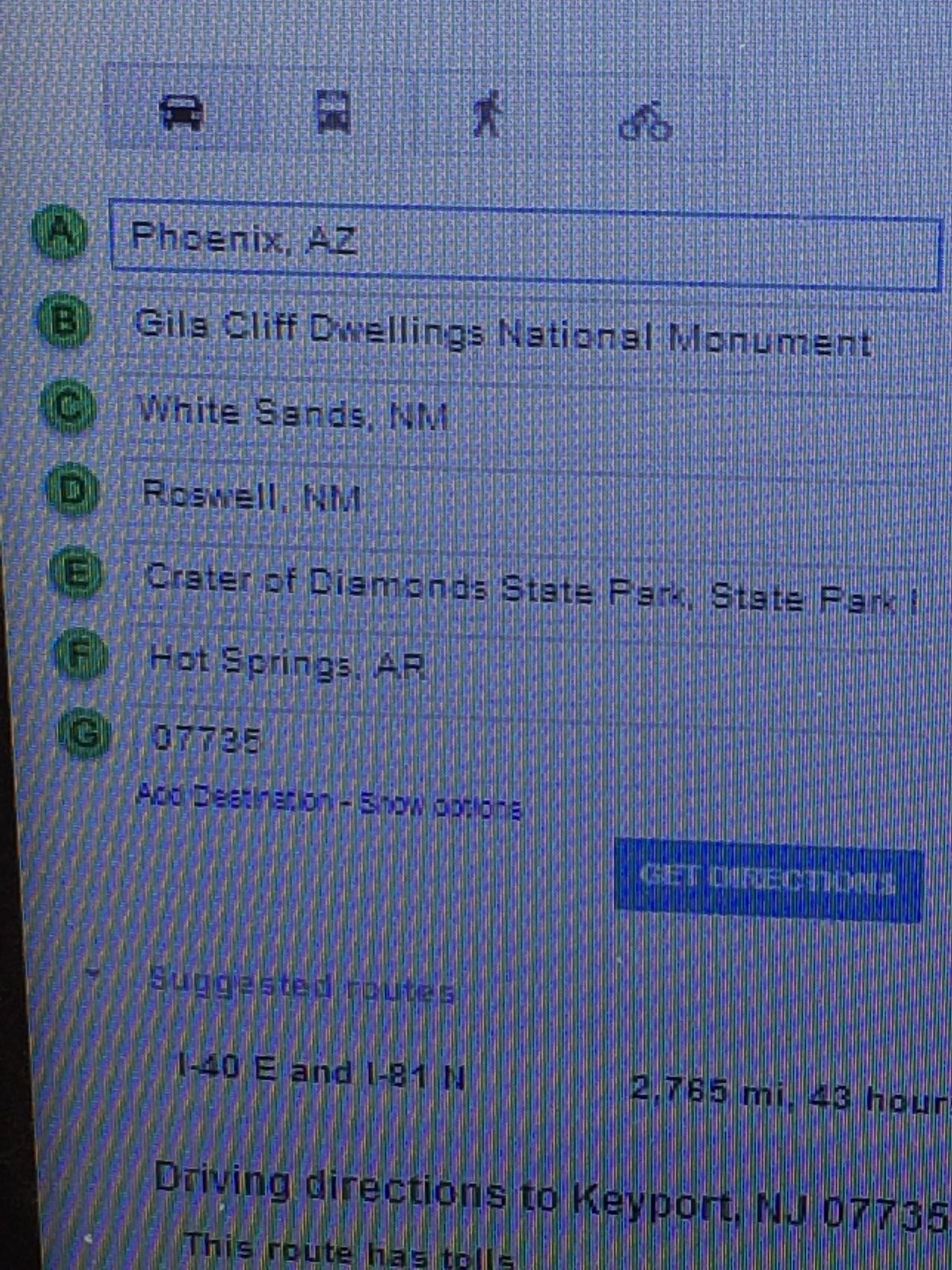This image features a pixelated photograph of a computer screen displaying navigational directions, which unmistakably highlights the individual pixels with a meringue-like texture interspersed with yellow and blue lines. The top portion of the screen showcases icons for different modes of transportation – a car, bus, pedestrian, and bicycle – with the car icon prominently highlighted in blue.

Beneath these icons, a vertical list of green circles labeled A through G outlines various destinations. The destinations listed next to these letters are: Phoenix, Arizona; Gila Cliff Dwellings National Monument; White Sands, New Mexico; Roswell, New Mexico; Crater of Diamonds State Park; and Hot Springs, Arkansas.

Following the destination list, the image details the routing information: "07735 Add Destination Show Options Get Directions Suggested Route, I-40 East and I-81 North, 2,765 miles, 43 hours, Driving Directions Keyport, NJ 07735." A notable caveat indicates the presence of tolls along this suggested route.

The juxtaposition of these navigational details against the pixelated background underscores the digital nature of the displayed directions, providing a comprehensive view of a long-distance driving route spanning multiple significant landmarks and ending at Keyport, New Jersey.